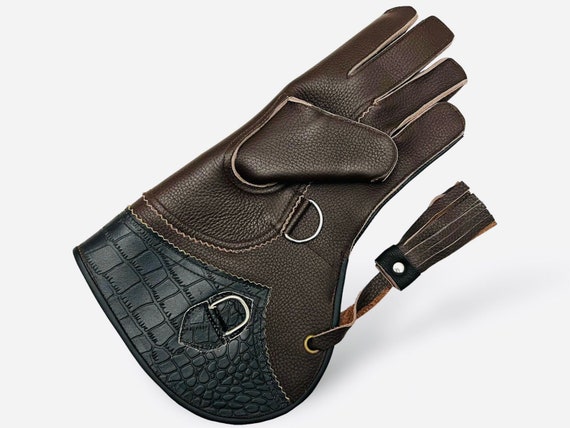In the image, there is a color photograph depicting a uniquely shaped leather glove in landscape orientation against a light gray background. The dark brown leather glove has thick, sturdy-looking fingers which point towards the top right corner of the image. The notably odd aspect of the glove is its elongated, bulbous wrist area, which flares out like a pouch or cuff and is covered in black material with a faux crocodile texture. Along the glove's body, there are detailed stitching and several metal embellishments, including a silver half buckle in the center of the palm and another silver buckle at the peak of a V-shaped stitching on the cuff. Below the thumb area, and along the wrist, small silver rings are attached. A leather tassel, hanging from a brass-riveted grommet, is attached on the right side of the cuff and points upward at an angle. This glove, possibly used by falcon trainers to protect themselves from the bird's talons, is depicted in a style of photographic realism and representational product photography.